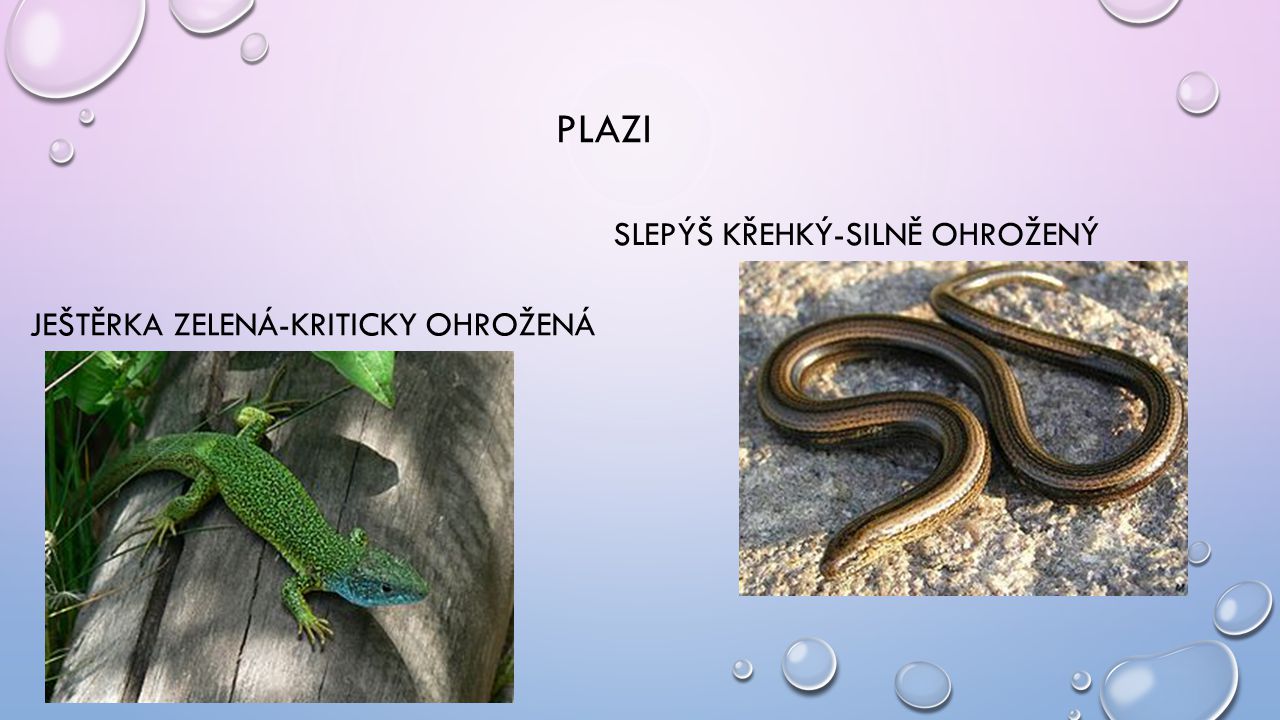This detailed image, resembling a PowerPoint slide, features the title "PLAZI" in bold capital letters centered at the top. The slide is framed with a pastel background transitioning from light lavender to deeper indigo hues, adorned with decorative bubbles or raindrops scattered across the surface. Two photographs dominate the slide: on the left, a vibrant green lizard, likely a gecko, is perched on a wooden log, while the right showcases a brown and white snake curled up on a stone slab. Accompanying these images is text in a European language, possibly Polish, adding an element of intrigue. The overall dimensions of the image are similar to a widescreen high-definition TV, emphasizing a wide rather than tall layout. The image captures a harmonious blend of nature-themed visuals and educational presentation, enriched with diverse colors including green, brown, and subtle pastel shades.